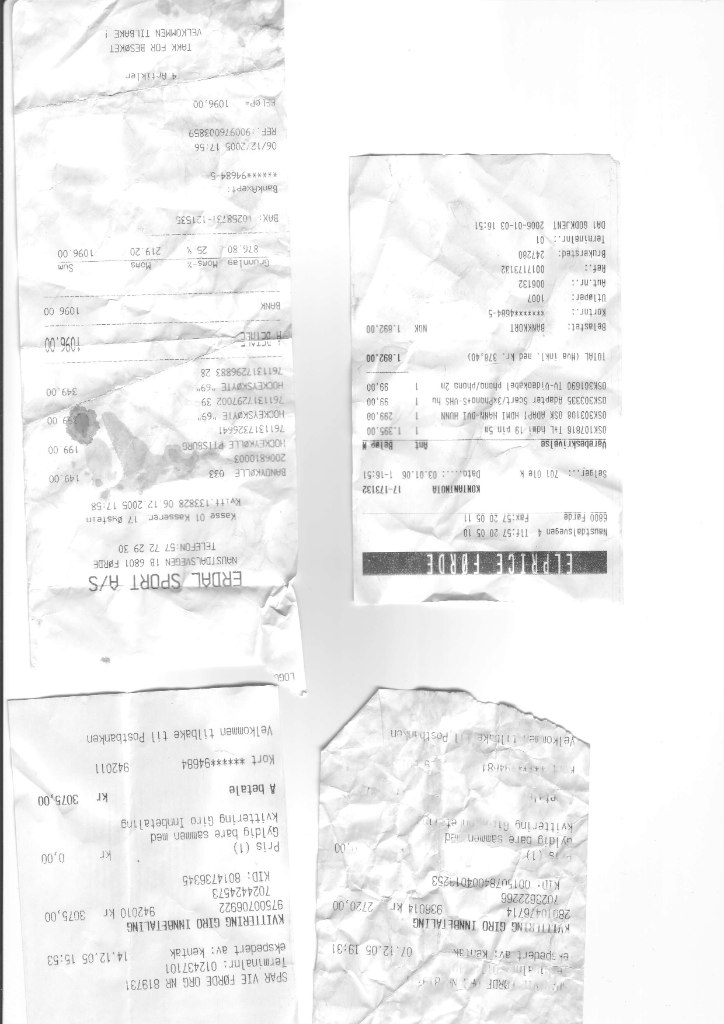This photograph captures four noticeably crumpled and poorly photocopied receipts, all displayed upside down. Each receipt is white, with visible shadow contrast created by the crinkles. The receipts are in a foreign currency denoted by "KR." Starting from the bottom right corner, there's a torn and folded receipt that's difficult to read. Above it, another crumpled receipt plainly shows "L. Price Ford" in black title text. In the bottom left of the image, an indiscernible receipt can be seen, with its top cut off in the photograph. Positioned above this, stretching the entire length of the image, is a particularly long and damaged receipt from "Erdahl Sport A/S," showing signs of significant wear, including possible spillage.